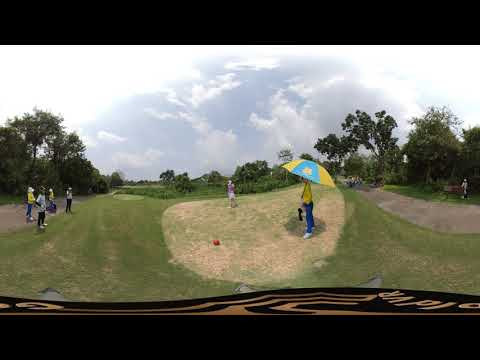This outdoor, daytime photograph, rectangular in shape with a black header and footer, captures a scene that appears to be on a golf course. The image itself is quite pixelated and blurry, but several details can still be discerned. The center of the photo is dominated by an individual standing on a grassy area, within a paler circle that appears sandier or drier, reminiscent of a golfing zone specifically cut out for play. This central figure is dressed in a yellow shirt and blue pants, holding a matching blue and yellow umbrella above their head.

To the left of this person stands another individual, seemingly mid-swing, possibly a golf player in action. Further left in the image, a group of four people can be seen, scattered along a path extending towards the horizon line. They appear to be wearing outfits complementing the central figure's clothing – two in yellow and blue and two in similar colors. On the far right, another person similarly dressed is visible, perhaps walking along a trail.

The scene is framed by a row of trees acting as a natural border, with a blue sky filled with white clouds above. On the far side of the hill in the lower portion of the photograph, a slight upward slope leads to another walking path and a distant bench. The presence of a red ball in the oval patch of mowed grass adds to the golf course ambiance. All these elements together craft a serene and detailed portrait of a day out on a golf course, despite the image's low resolution.